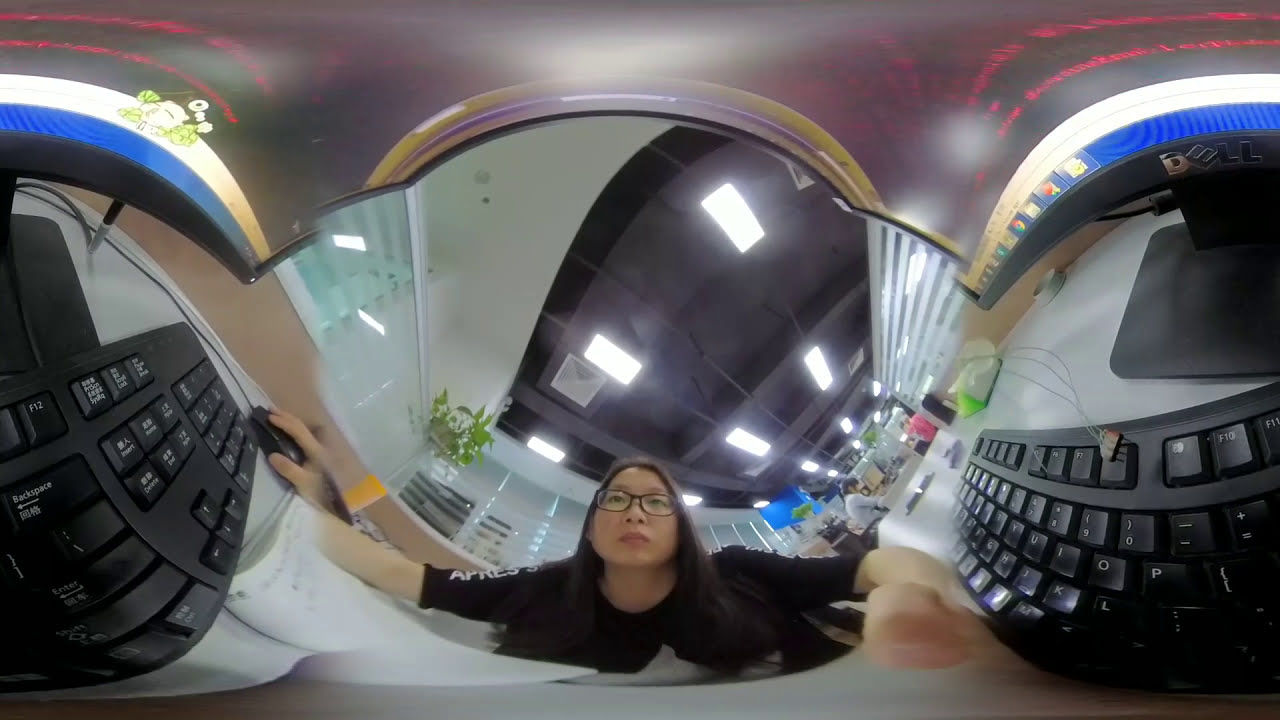The image is a composite of three distinct scenes encapsulated within bubble shapes. The central bubble features a girl with straight black hair, wearing glasses and a black shirt, looking slightly upwards. Behind her, there is an interior setting with white walls and visible ceiling lights, suggesting it might be a room, cafe, or office space. The left bubble captures a black keyboard with a hand using a mouse, while the right bubble shows another black keyboard, a monitor with a pinkish top hue, blue and white borders, and a black border labeled "Dell." The overall composition is surrounded by a thumbnail icon that typically represents a failed-to-load image. This icon is a tiny square with a dog-eared upper right corner, a white circle on a blue background in the upper left, a vaguely green area in the lower left, and a white diagonal bar running from the center bottom to the center right edge.